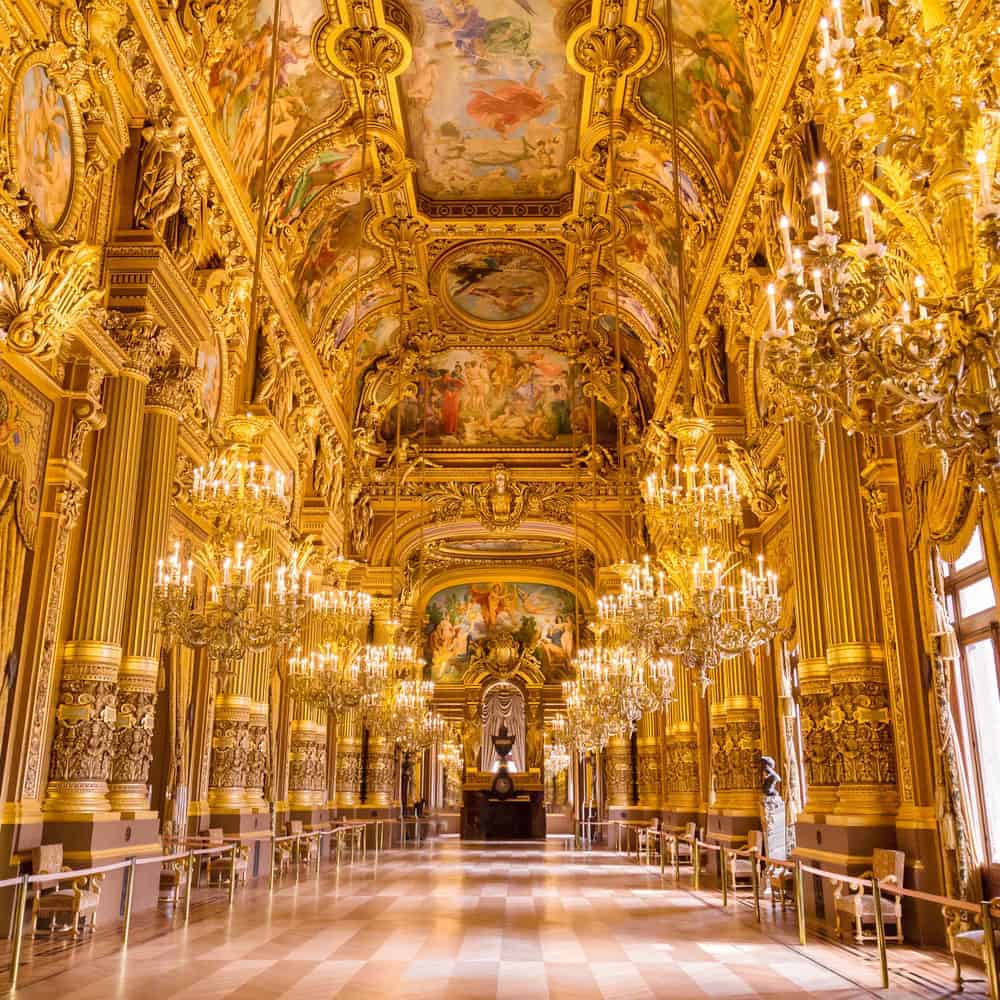This image captures the grandiose interior of an ornately designed hall, which could be part of a castle, church, or museum. The entire space is bathed in a golden hue, with walls and structures adorned in what seems to resemble gold. The floor is an elegant checkerboard pattern of shiny marble tiles. Ornate chandeliers hang from the ceiling, numbering around 15 on each side, casting a majestic glow throughout the space.

The ceiling is adorned with exquisite frescoes and murals, reminiscent of Renaissance paintings, creating an awe-inspiring vista above. The architectural design features impressive Doric columns that stretch from the floor to the ceiling, which is approximately a hundred feet high. There are also numerous candlestick holders along the sides of the walls, each holding several lit candles that add to the ambient lighting.

At the end of the corridor, there is an object placed on a stand, though its exact nature is unclear. On the lower left-hand side of the hall, a person can be seen, adding a sense of scale to the grandeur of the hall. The windows along the sides allow for additional natural light to filter through, enhancing the opulent feel of the interior. This hall is a stunning example of architectural and artistic excellence, epitomizing luxurious design and intricate decorative elements.